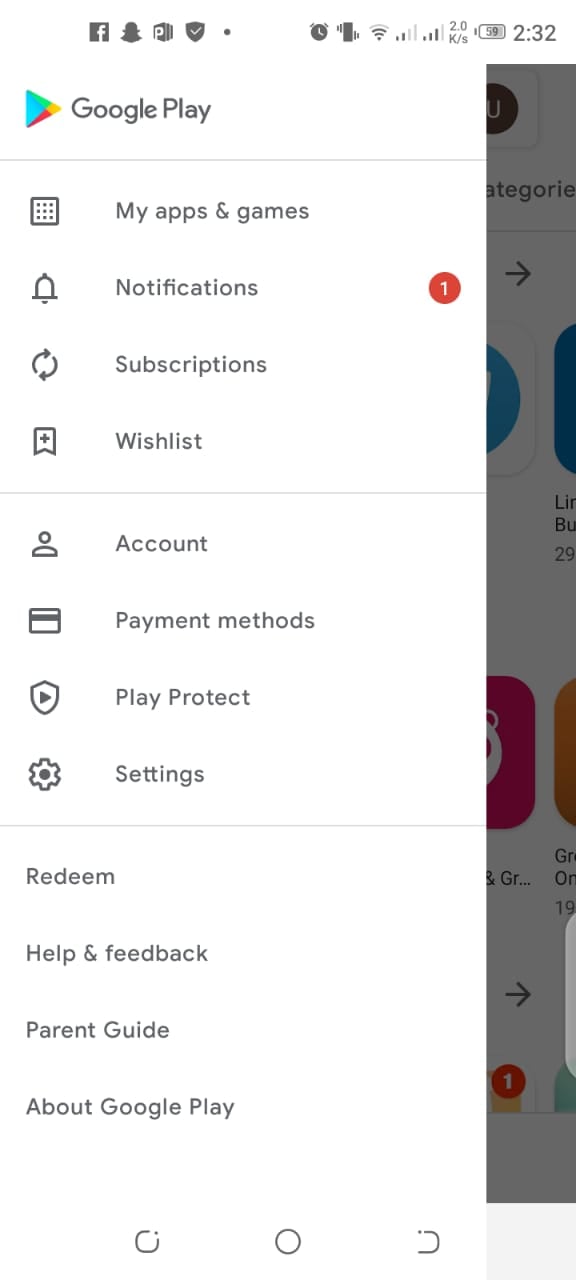This screenshot from a phone captures the Google Play interface, prominently displaying the current time at 2:32 and a partially filled battery icon at 90%, indicating the device is charging. The screen, which has a white background, is divided by several gray lines into distinct sections. 

At the top, the header of the Google Play app includes a small grid icon, labeled "My Apps & Games," adjacent to a bell icon with a red notification circle displaying the number '1', indicating one new notification. 

Below this is the "Subscriptions" section, followed by "Wishlist." The subsequent sections include "Account" with a credit card icon next to "Payment Method," "Play Protect," and "Settings." Further down are options labeled "Online," "Redeem," "Help and Feedback," "Parent Guide," and the final option "About Google Play." 

The bottom of the screen features the navigation bar, which includes a central circular home button flanked by the typical Android navigation icons.